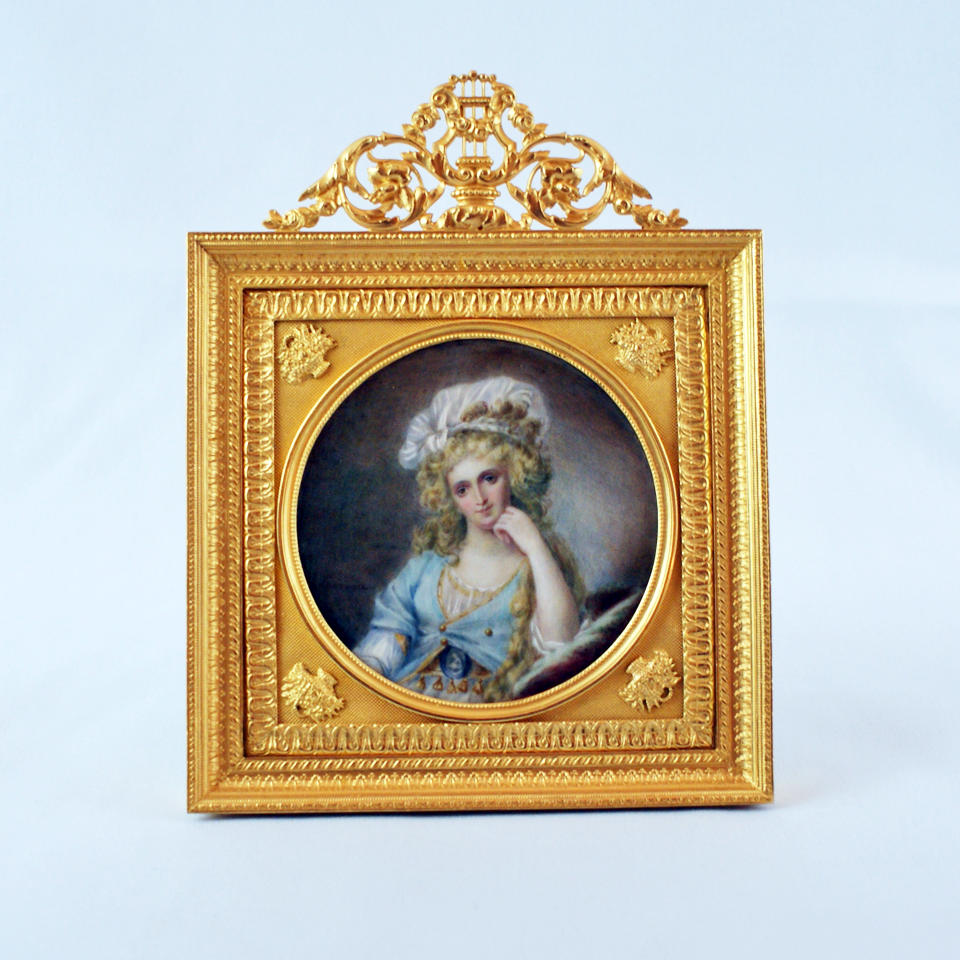The image is a historical painting of a regal woman, housed in an antique, gold frame with elaborate floral patterns on all sides. At the top of the square frame, there's a crown-like ornamentation, also in gold, adding to its ornate design, along with additional golden insignias in the corners. The central focus is a circular oval medallion portraying a white woman with blonde, curly hair that cascades down her left shoulder, part of which is tucked under a white bonnet cap adorned with feathers. She is dressed in a baby blue, almost cyan, button-up overcoat with quarter sleeves and gold trim over a white gown. Her posture is relaxed and serene, with her right arm bent at the elbow, supporting her chin on her folded fingers, and her head slightly cocked to the left. The backdrop of the entire composition is a light blue, enhancing the allure of the golden frame and the portrait it encases.